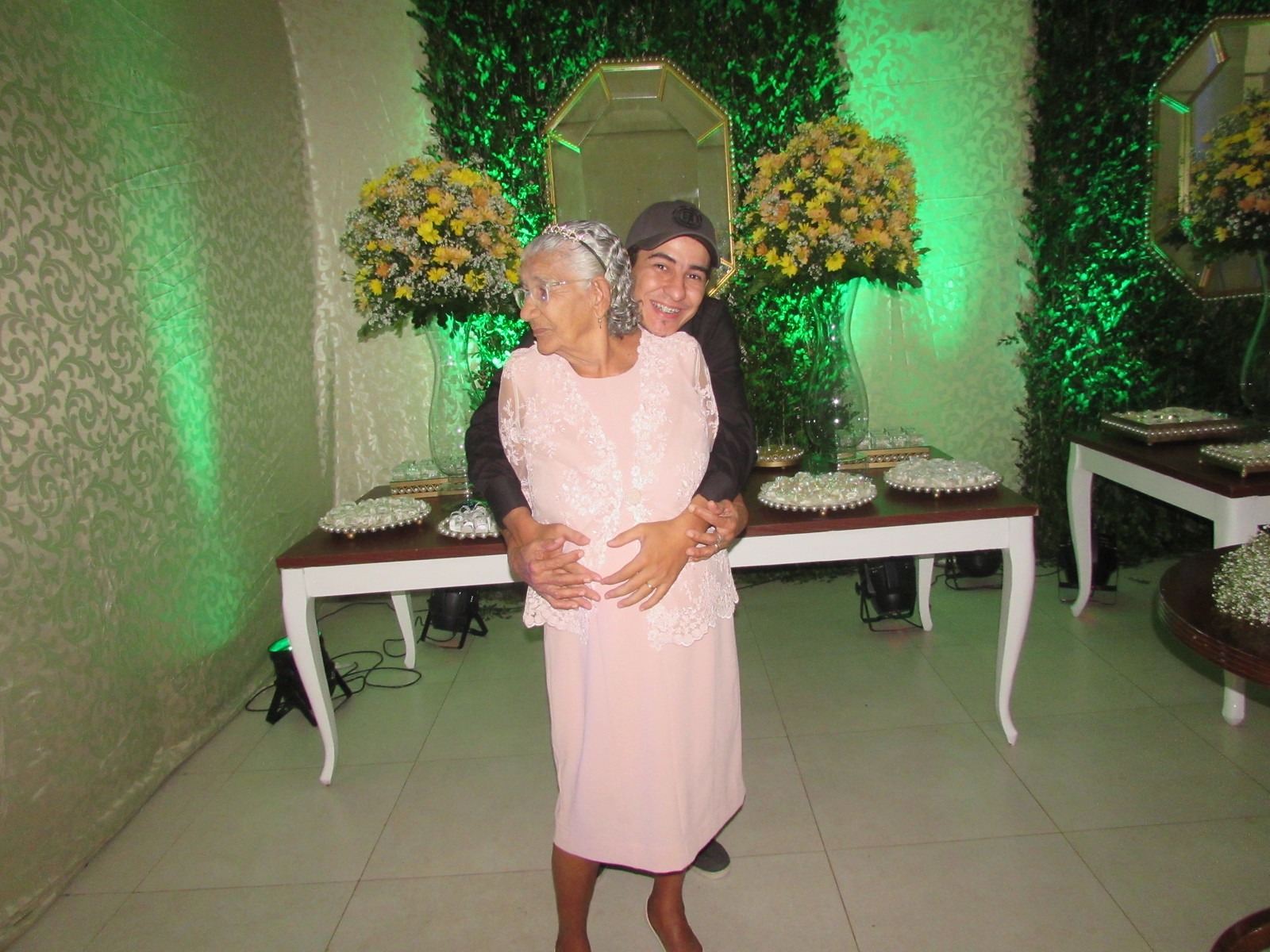The image captures an indoor celebration party with elegant decor and a festive atmosphere. Central to the photograph is an elderly woman with light brown skin, possibly of Mexican descent. She has silver-gray hair styled back and adorned with a delicate pink headpiece resembling a narrow tiara. She wears glasses and a light pink dress topped with a white lace jacket. The woman gazes off to the side while being hugged from behind by a young man, likely a teenager, who has light brown skin and wears a gray baseball cap and a long-sleeved black shirt. His arms are lovingly wrapped around her, and he is smiling directly at the camera.

The background features several tables with brown tops and white legs, adorned with various cream-topped pies and pastries. Large vases filled with yellow and orange flowers, complemented by greenery, add to the decor. The walls of the room have a pale, shiny metallic wallpaper with a repeating vine pattern, and green spotlights enhance the festive ambiance. The floor is lined with large white square tiles, completing the elegant setting.